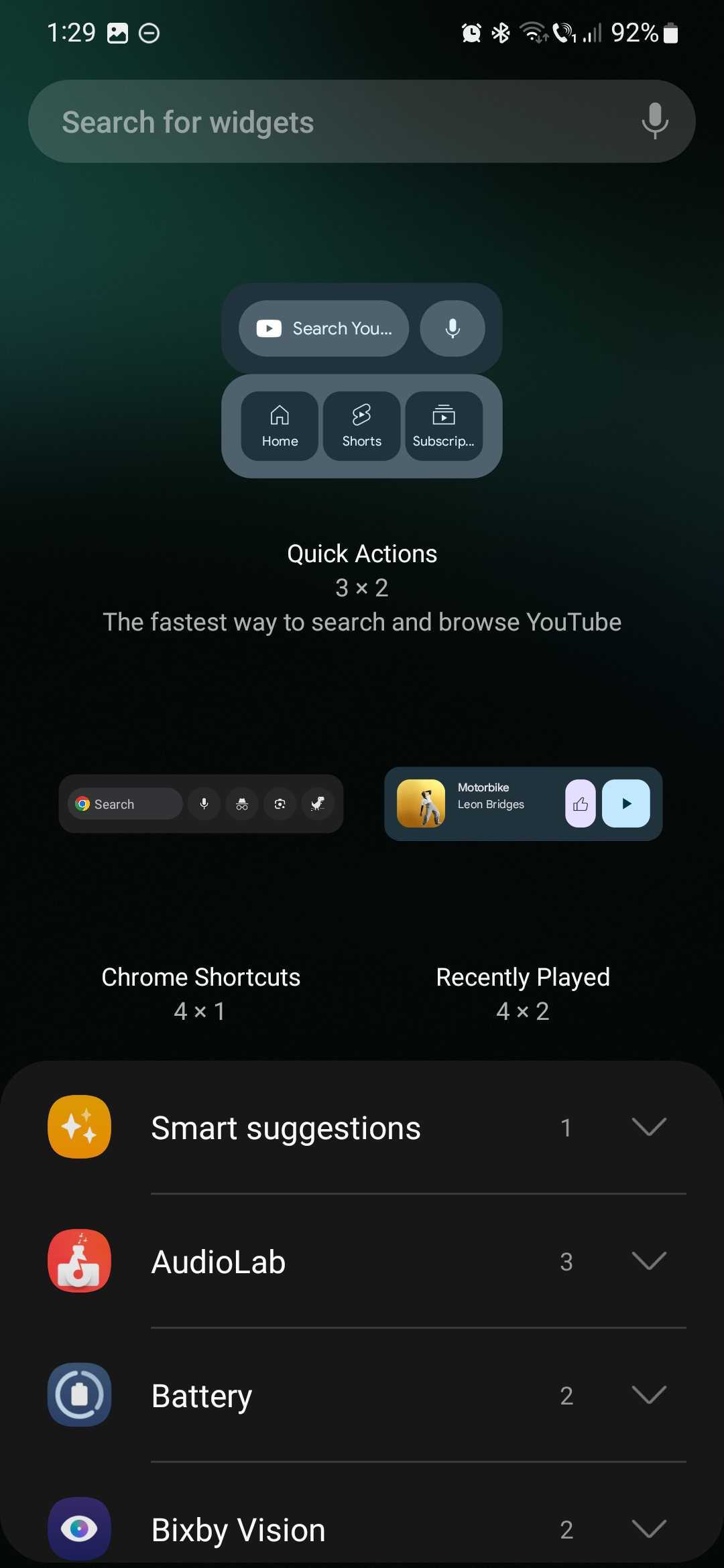A detailed screenshot image, likely captured from a smartphone, showing a variety of interface elements:

In the top-left corner, the status bar displays "1:29" followed by an icon and a circular icon with a minus sign. On the top right, there are several status icons: a clock, Bluetooth, and Wi-Fi (with two bars filled), followed by a phone icon and signal bars indicating two bars of reception. Adjacent to these is a "92%" battery indicator with a battery icon.

Below the status bar, a long oval search bar reads "Search for widgets," with a microphone icon on its right side. Below this search bar are quick action buttons for YouTube: "Home," "Shorts," and "Subscriptions." A text string below these buttons reads "Quick Actions 3x2, the fastest way to search and browse YouTube."

Further down, a section labeled "Search" is visible, though the text appears small, followed by various icons. There is a user profile picture and two labeled buttons: "Shortcuts 4x1" and "Recently played 4x2."

At the bottom, four selectable options with corresponding icons and dropdown arrows are listed: "Smart Suggestions," "Autolab," "Battery," and "Bixby Vision," each with associated numbers.